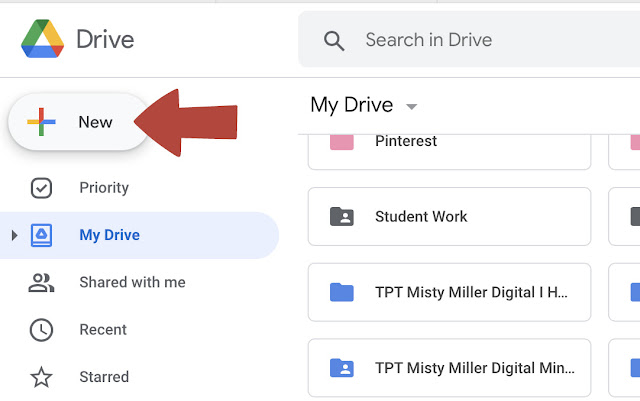In this image, we see the interface of Google Drive. In the upper left corner, the recognizable Google Drive logo is displayed, composed of a green, yellow, blue, and red triangle, accompanied by the text "Drive." To the immediate right of this, a gray search bar featuring a magnifying glass icon displays the placeholder text "Search in Drive," indicating the search functionality, though no query is entered.

Further down the page, a prominent red arrow points towards a button labeled "New." This button is distinguished by a colorful plus sign reflecting Google's iconic colors. The red arrow emphasizes the importance of this button, likely suggesting to users that they should click it to create new content.

Below this section, there are several organizational headings: "Priority," "My Drive" (highlighted in blue), "Shared with me," "Recent," and "Starred." On the right side, there's another "My Drive" section with a downward-facing gray arrow. Additionally, this section contains several folders: "Pinterest" (marked with a pink folder icon), "Student Work" (marked with a black folder icon), and two instances of "TPT, Misty Miller Digital" (each marked with a blue folder icon).

The background of the page is a plain white, with various sections and elements neatly arranged and distinguished by subtle borders and icons, exemplifying the clean, minimalistic design typical of Google's suite of applications.